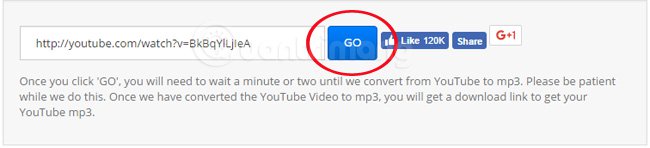The image displays a screenshot of step-by-step instructions for sharing or copying a link. The instructions are presented within a small, gray rectangular box containing a smaller white rectangle with an explicit text link: http.youtube.com, designated for a specific video. Adjacent to this white box, there's a prominent blue rectangular "Go" button encircled in red, likely indicating the need to press it.

To the right of the "Go" button, there are two smaller, darker blue rectangular buttons: one with a thumbs-up icon for liking the post on Facebook, and another featuring a share icon. Further to the right, there's one final, even smaller button with a white background and red text, suggesting an action related to Google Plus.

Beneath these elements, in a single line, dark gray text explains: "Once you click Go, you will need to wait a minute or two until we convert from YouTube to MP3. Please be patient while we do this. Once we have converted the YouTube video to MP3, you will get a download link to get your YouTube MP3." No further information is displayed in the image.